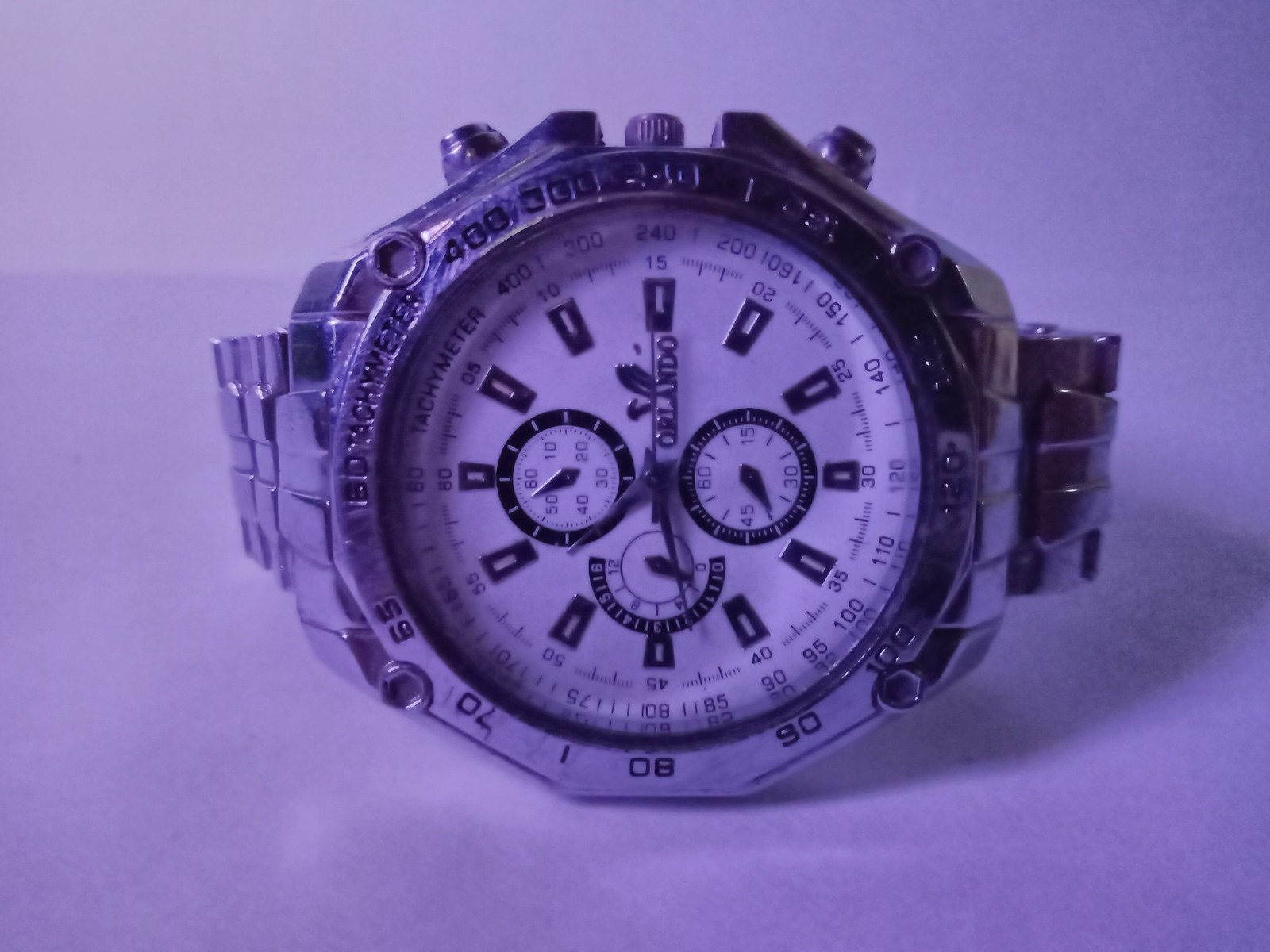This image shows a detailed side view of a wristwatch, prominently made of metal with a completely silver band and casing. The watch is positioned on its side around the nine o'clock mark. The face of the watch features a white background with black markers, though it notably lacks numerical hour markers, which complicates time-telling at a glance. The watch is a chronograph, equipped with three sub-dials possibly used for various timing functions: one at twelve o'clock likely for seconds, one at six o'clock which could be another second or minute timer, and one at nine o'clock that seems to mark hours or half-hours. Surrounding the face is a tachymeter scale with numbers ranging from 400 to 60. The watch's three crowns include a central knob for adjusting the time and additional buttons on either side for operating the chronograph functions. Although the brand name, 'Odelaldo,' is inscribed on the right side of the face, it does not resonate with the observers.